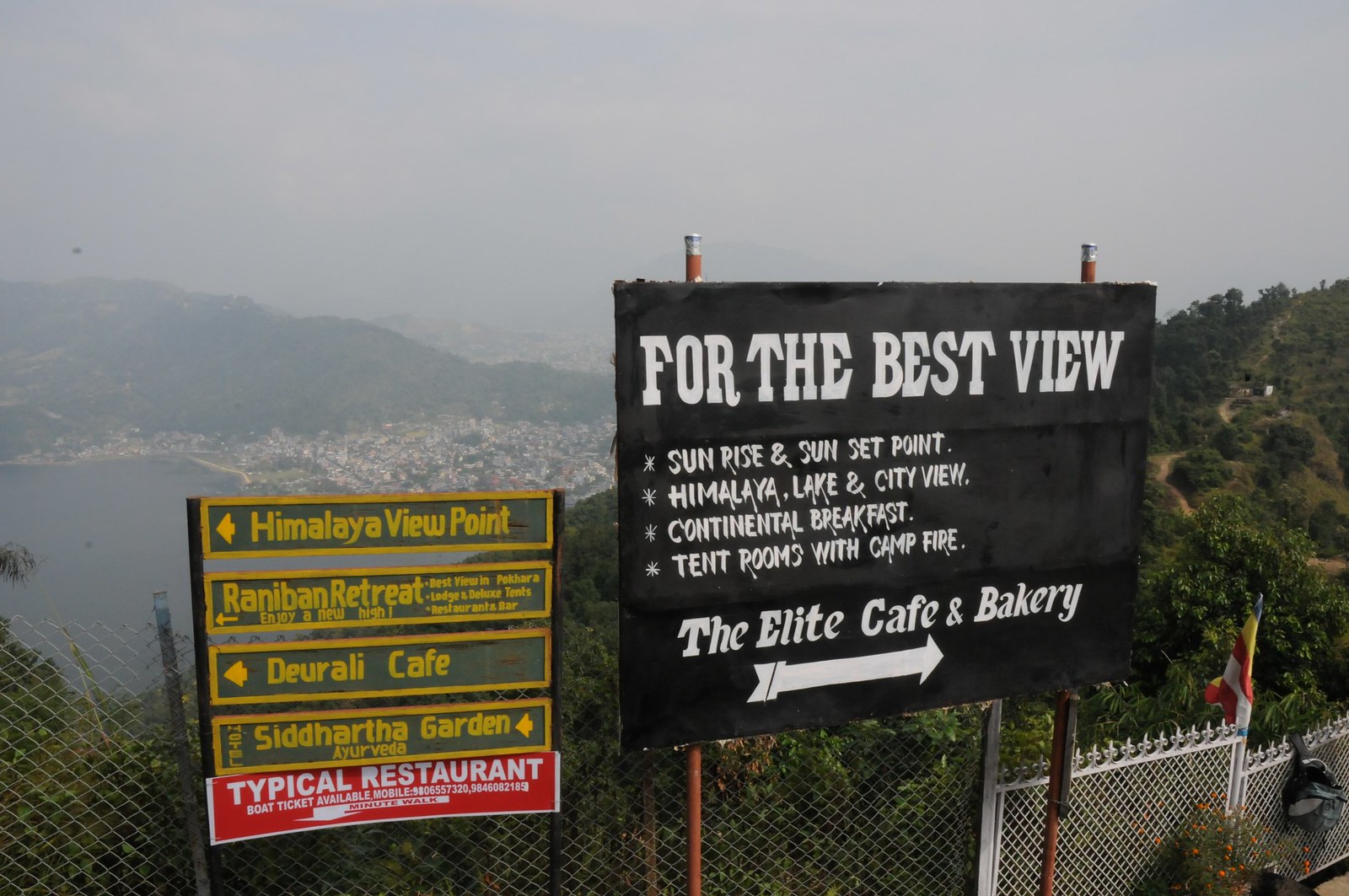This photograph captures a picturesque viewing point situated on the side of a mountain. In the foreground, there are two signposts surrounded by a lush green landscape, a bay, and a populous city in the distance, beneath a gray, foggy sky.

The signpost on the left features a series of yellow directional signs pointing to the left. The top sign says "Himalaya Viewpoint," followed by "Rannaban Retreat" with the slogan "Enjoy a new high," and then "Deurali Cafe." Below these, another sign directs towards "Siddhartha Garden," with "Araveda" mentioned next to it. At the bottom, a distinctive red and white sign reads "Typical Restaurant" and notes "Boat Tickets Available, Mobile" with phone numbers, along with "Minute Walk" and an arrow.

On the right, a black sign with white text promotes several attractions: "For the Best View, Sunrise and Sunset Point, Himalaya, Lake and City View, Continental Breakfast, Tent Room with Campfire," and directs towards "The Elite Cafe and Bakery" with an arrow. In the background, a chain-link fence encloses the area, beyond which stretches a serene mountain range, verdant with trees, a large expanse of blue water, and the distant cityscape.